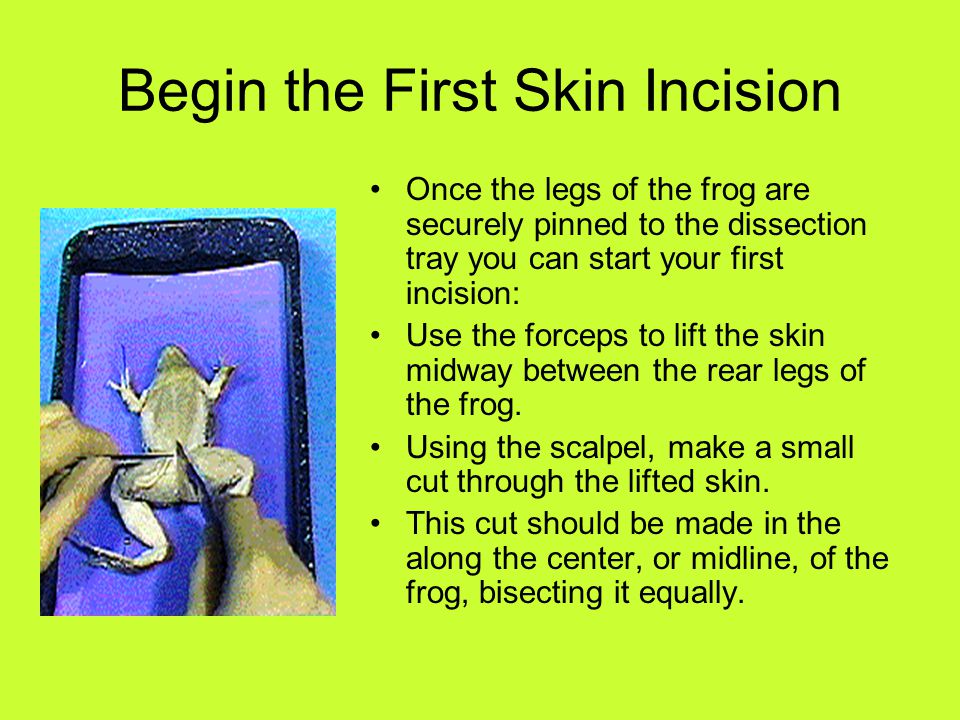The slide presents an educational guide on the initial steps of dissecting a frog, aimed at facilitating an anatomical study. Dominating the slide is a detailed instructional text on making the first skin incision. It reads: "Begin the first skin incision. Once the legs of the frog are securely pinned to the dissection tray, you can start your first incision. Use the forceps to lift the skin midway between the rear legs of the frog. Using the scalpel, make a small cut through the lifted skin. This cut should be made along the center or midline of the frog, bisecting it equally." The left side of the slide features a photograph illustrating the described procedure. In the photograph, a gloved hand holds a pair of tweezers and a scalpel as it carefully makes the initial incision on the frog’s belly, which is pinned down on a black dissection tray lined with a blue paper towel. The tray is placed on a blue surface. The background of the slide is a striking neon green, creating a clear contrast with the black text and highlighting the instructional content. The overall setting suggests that this slide is part of a PowerPoint presentation used for educational purposes, likely in a biology or anatomy class.